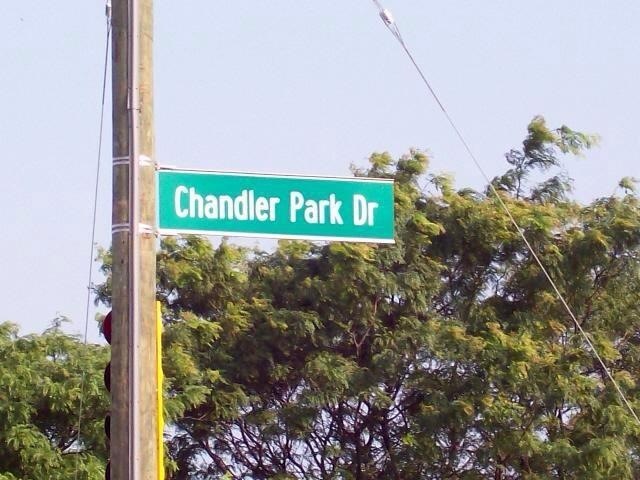A wooden utility pole, mounted with a heavy conduit on the side facing the camera and a wire guidance attached for support, dominates the foreground of this image. Affixed to the pole is a green, rectangular street sign with white text reading "Chandler Park Drive." The background features a lush tree with long, flowing green leaves that stretches from the lower left corner to the center right side of the horizontal frame. Above this verdant backdrop, the sky manifests as a solid yet pale blue, providing a serene contrast to the detailed textures of the pole and foliage.